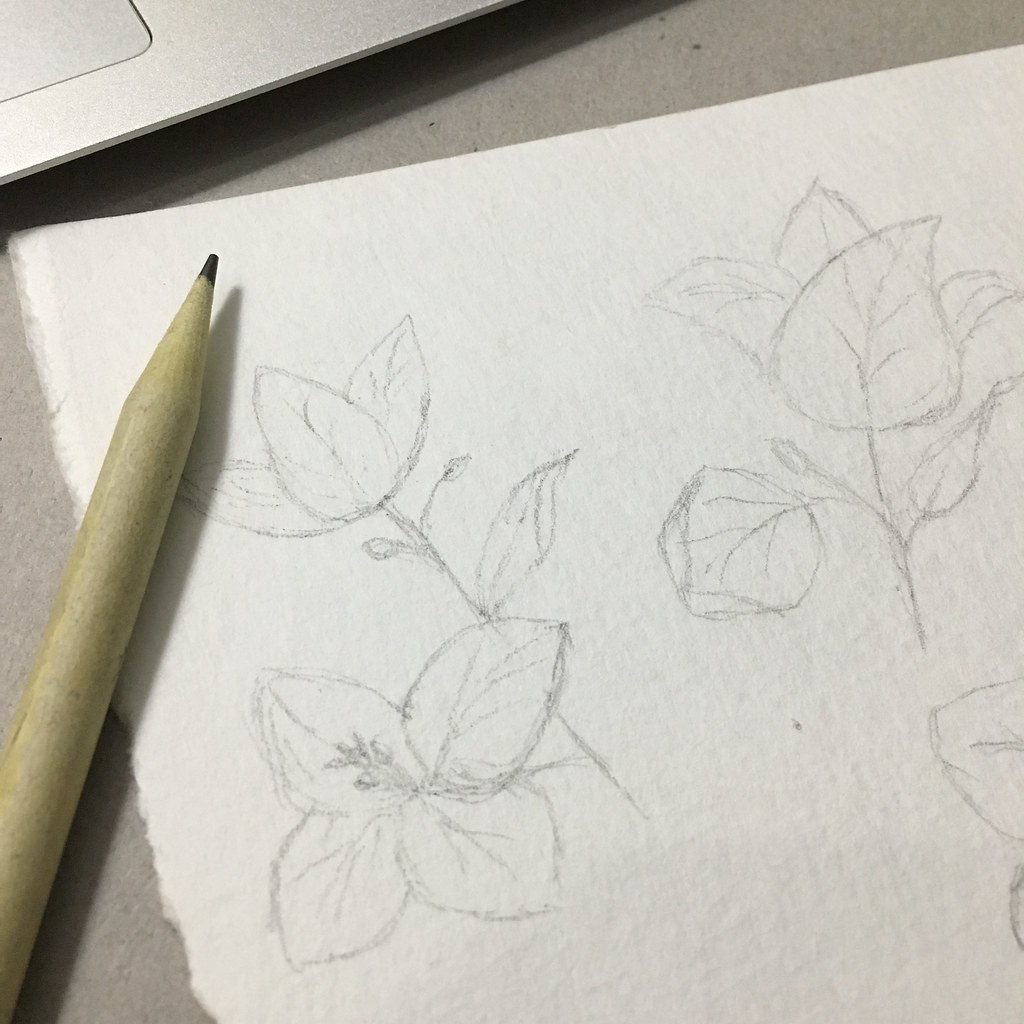This image captures an angled view of a partially visible piece of paper, featuring two pencil-sketched flowers. On the left side of the paper, there are two views of a four-petaled flower—one from the top and the other from the side. Each petal is meticulously outlined in pencil, with detailed shading highlighting the flower’s pistils that emerge prominently from the center. The flower has a single leaf to the right, rendered with fine, deliberate strokes.

To the right side of the paper, another flower sketch is depicted, characterized by large, tear-drop-shaped leaves. This flower’s petal arcs gracefully downward to the left, with the edges intricately curved inward, adding depth and texture to the sketch, all drawn in pencil with careful attention to detail.

In the left side of the photo, a pencil is visible, placed at an angle on the gray table. The pencil's top parts overlap slightly with the left corner of the sketch paper, hinting at the artist’s ongoing work. In the top left corner of the image, a portion of the bottom of a silver laptop is visible, with a glimpse of the silver trackpad adding a modern contrast to the classic, hand-drawn sketches.